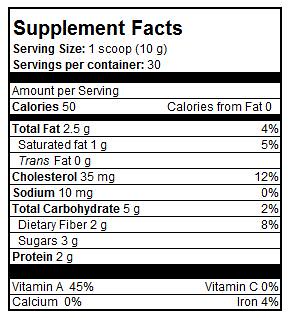This image depicts a detailed supplement facts label for a dietary supplement. The label specifies a serving size of 1 scoop or 10 grams, with 30 servings per container. Each serving contains 50 calories, with zero calories from fat. The total fat content per serving is 2.5 grams (4% of the daily value), including 1 gram of saturated fat (5% daily value) and 0 grams of trans fat. It also lists 35 milligrams of cholesterol (12% daily value), 10 milligrams of sodium (0% daily value), 5 grams of total carbohydrates (2% daily value), which includes 2 grams of dietary fiber (8% daily value) and 3 grams of sugar. Additionally, each serving provides 2 grams of protein. The vitamin content includes 45% of the recommended daily intake for vitamin A, 0% for vitamin C, 0% for calcium, and 4% for iron.